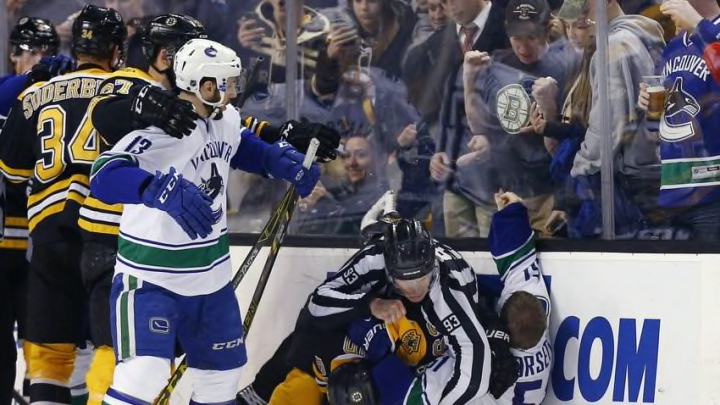The photograph captures a dynamic and intense moment in a hockey game, centered around a fight between players. The scene is dominated by a referee attempting to separate two opposing players—one in a black and gold uniform and the other in a blue and white Vancouver jersey. The action unfolds on the left-hand side, where two players in black and gold are restraining a Vancouver player, suggesting the fight could escalate. Behind this chaotic tableau, players are seen converging, indicating potential further conflict. The image is set against a backdrop of an energetic crowd, visible through the clear barrier of the rink. Fans, clad in diverse attire ranging from casual t-shirts to suits and sports jerseys, are animatedly cheering, with one even holding a beer. Notably, a player with the name "Sod" and the number 34 is identifiable among the blue and white-clad Vancouver team, adding specificity to the frenzied scene.